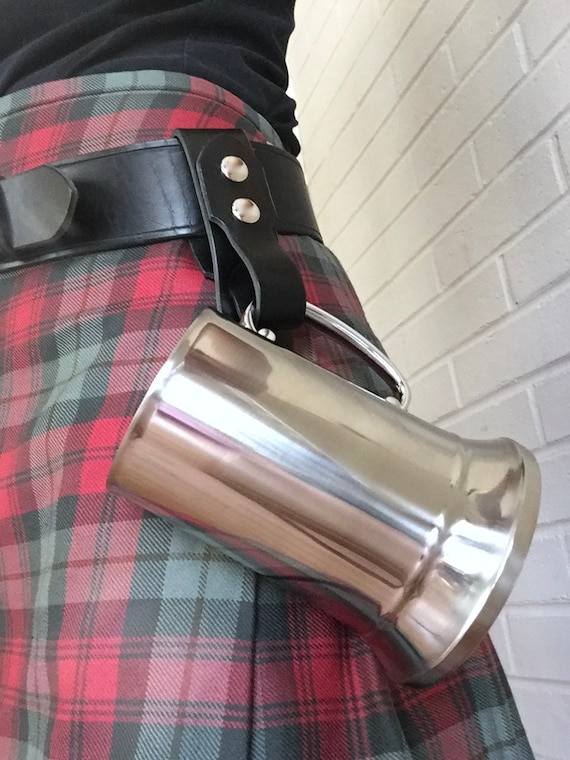This is a detailed color photograph showcasing an angled view of a woman's waist, set against a whitewashed brick wall. The woman, dressed in a black shirt, has her lower torso and waist prominent in the image. She is wearing a red and green plaid skirt which is secured by a wide leather belt, adorned with two silver studs. Dangling from a leather loop on the belt is a large, shiny silver beer mug, attached by its handle. The beer mug is highly reflective, capturing light from a nearby window. The woman's thin frame is subtly noticeable beneath her clothing. The white bricks in the background are arranged diagonally, adding texture and depth to the scene.